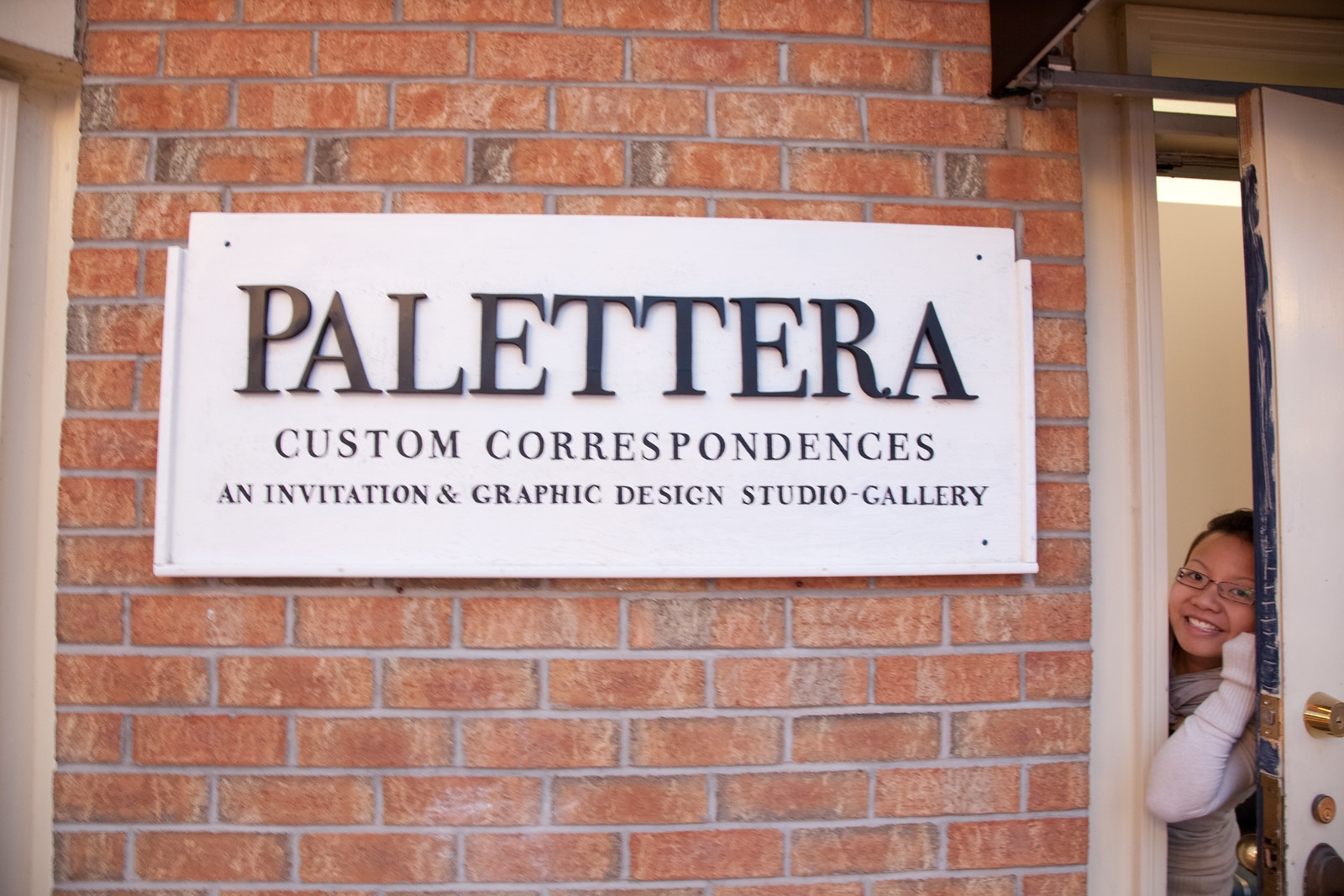This detailed photograph captures the exterior of a business establishment with a clean, newish red brick wall. Prominently displayed on the wall is a large, rectangular white plaque that reads "Palaterra" in bold black letters, followed by "Custom Correspondence an Invitation and Graphic Design Studio Gallery" beneath it. To the right of the plaque, a cream-colored door with matching trim is slightly ajar, revealing a young Asian woman with black hair pulled back, wearing small rimless glasses, and a long-sleeved gray top. She is holding the door open about a foot and peeking out with a broad smile, directly engaging with the camera. Inside the slightly open door, a beige wall and some fluorescent tube lighting are visible, suggesting a welcoming and well-lit interior space.